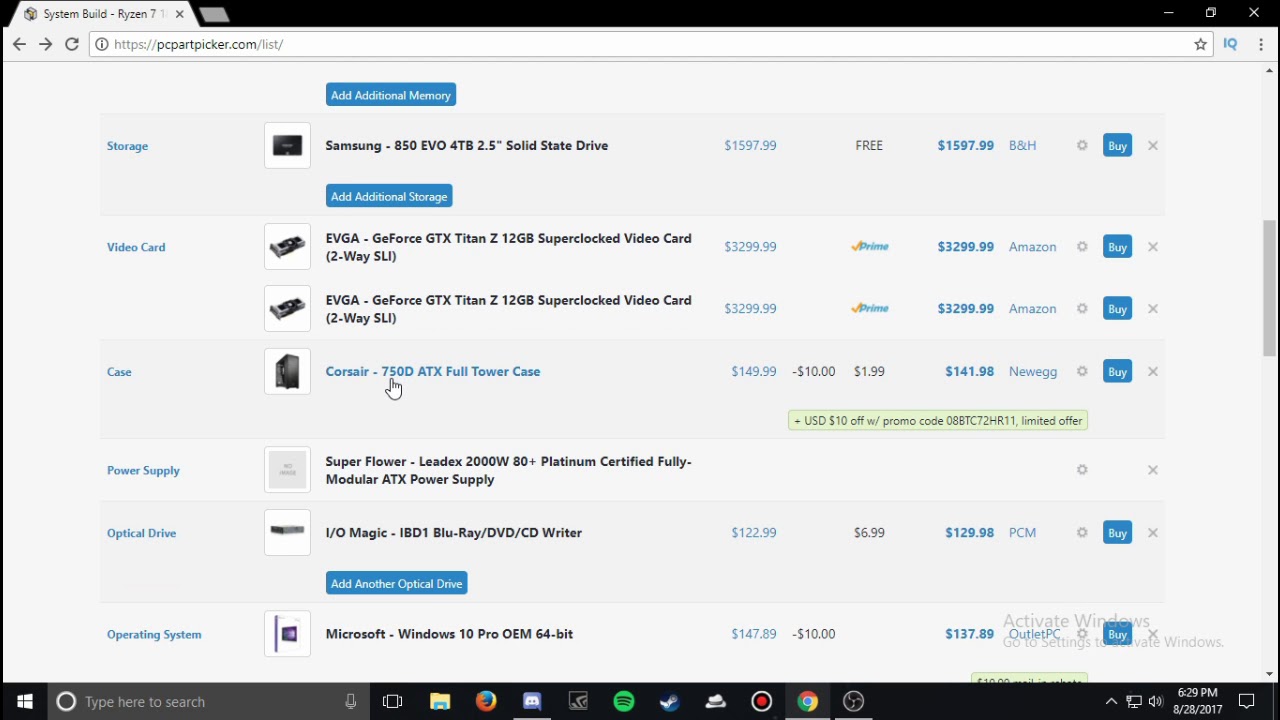Image Caption:

The image depicts a search interface on an electronic system parts website. At the top, there is a search bar with the query "system build razor." Below the search bar, a list of various computer components is displayed, including options for storage, video card, courier, power supply, optical drive, and operating systems. The first item listed is the "Samsung 850 EVO 40BS Solid-State Drive," followed by another entry marked as "EV." The third item appears to be a duplicate or similar to the second entry. Each component is accompanied by its respective price. The layout appears cluttered and somewhat confusing, making it difficult to navigate through the technical items.